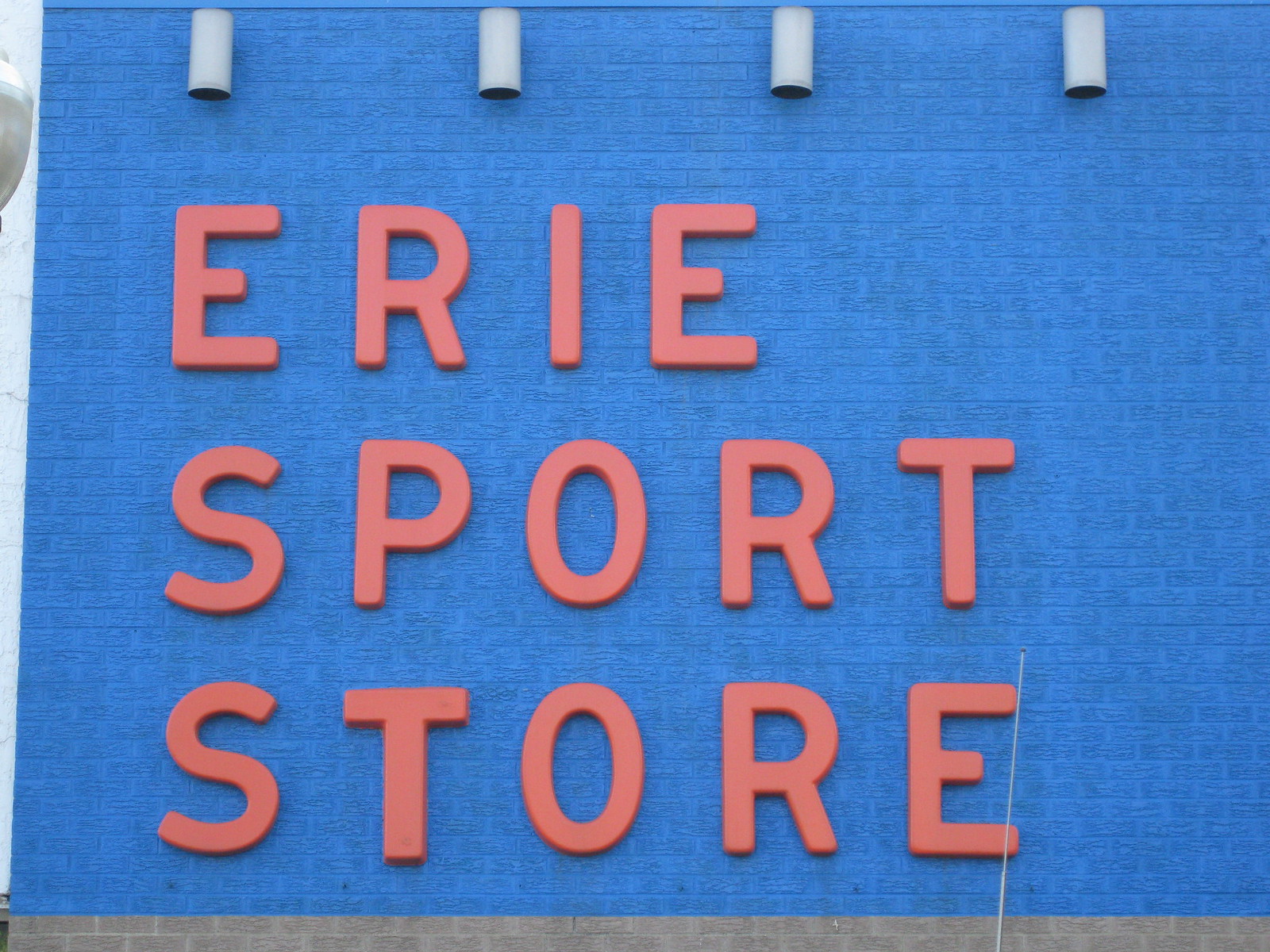The photograph captures a blue brick-walled building that dominates the frame. Along the bottom of the image, a slim strip of grey-painted brick is visible, contrasting the blue wall, while a thin strip of white sky is seen on the left side. Mounted evenly along the upper edge of the building are four grey cylindrical fixtures with black interiors, likely lights that are currently off due to the daylight. The name of the establishment, "Erie Sport Store," is prominently displayed in simple, all-caps, orange letters. The text is organized in three left-aligned lines: "ERIE" on the top line, "SPORT" on the second, and "STORE" on the third. This clear and straightforward sign stands out against the blue background, making the store easily identifiable.